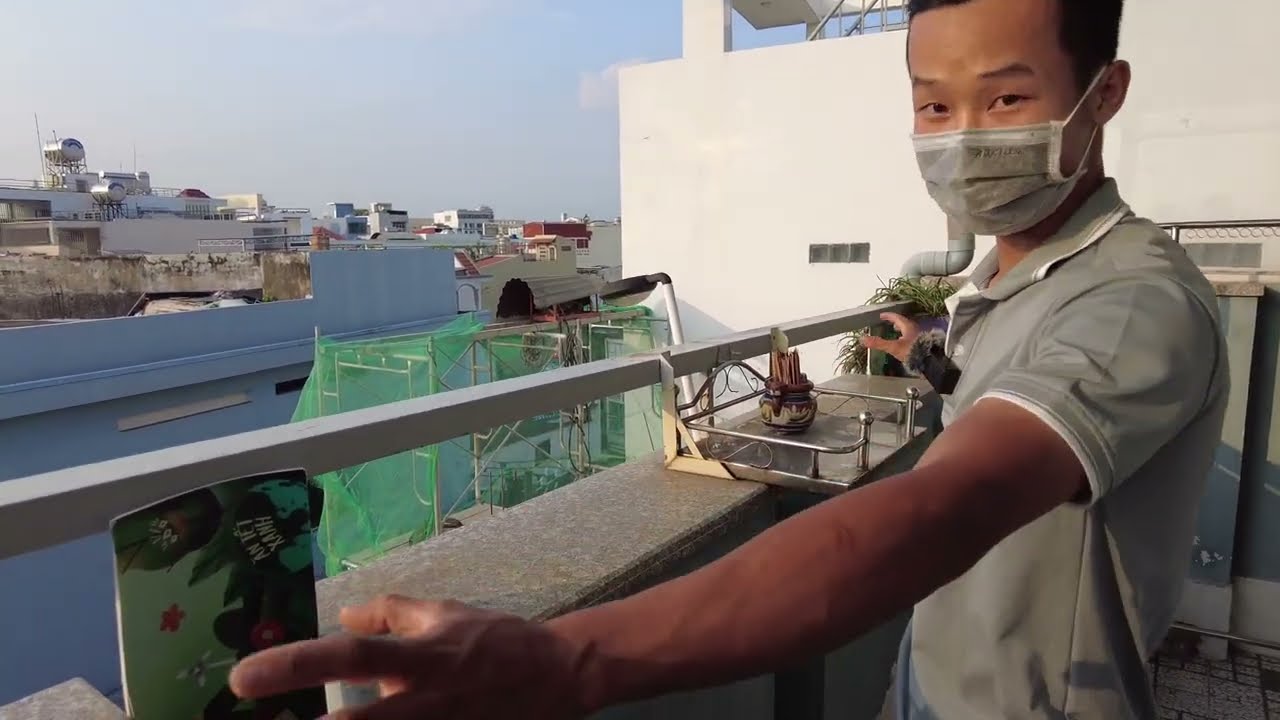This photograph captures an Asian man, seemingly in his mid to late 20s, standing on a balcony with a granite-topped ledge that features a metal railing. The man is wearing a gray polo shirt with white trim around the collar and sleeves, and a gray surgical mask, indicative of the COVID-19 period. He is looking directly at the camera, with one arm stretched out to the side, touching or hovering near the railing. In front of him on the ledge is a silver tray holding a little brown ceramic pot filled with coffee stirs. The background reveals an industrial-looking scene with a collection of buildings or possibly a large ship, characterized by a light gray color and various structures on it. Additionally, there's noticeable scaffolding with green netting. The sky above is blue with hazy clouds, indicating a sunny day. The image is taken from a close perspective, almost like a selfie, capturing the detail of the man's short black hair and the serene, yet industrial, setting around him.